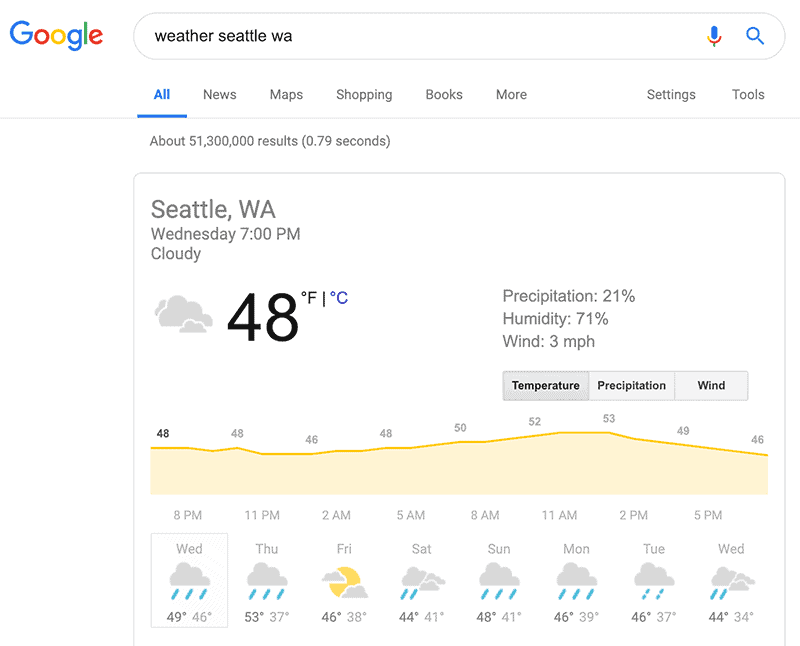This is a detailed screenshot of Google search results. The background is predominantly white in the upper left corner, featuring the iconic Google logo composed of alternating colors—blue, red, yellow, blue, green, and red. To the right of the logo is the search field displaying the query "weather Seattle, WA." Adjacent to this field are a microphone icon and a magnifying glass icon representing voice search and the search function, respectively.

Below the search bar, there is a navigation menu with various options: "All," "News," "Maps," "Shopping," "Books," "More," "Settings," and "Tools." The "All" tab is currently selected. In gray font just beneath this menu, the results information states: "About 51,300,000 results in 0.79 seconds."

Further down the page, a weather information box is prominently displayed. The top left of the box indicates "Seattle, WA," followed by "Wednesday 7 p.m. Cloudy." An icon of a cloud is shown alongside the text "48°F." Additional weather details include a precipitation rate of 21%, humidity at 71%, and wind speeds of 3 miles per hour.